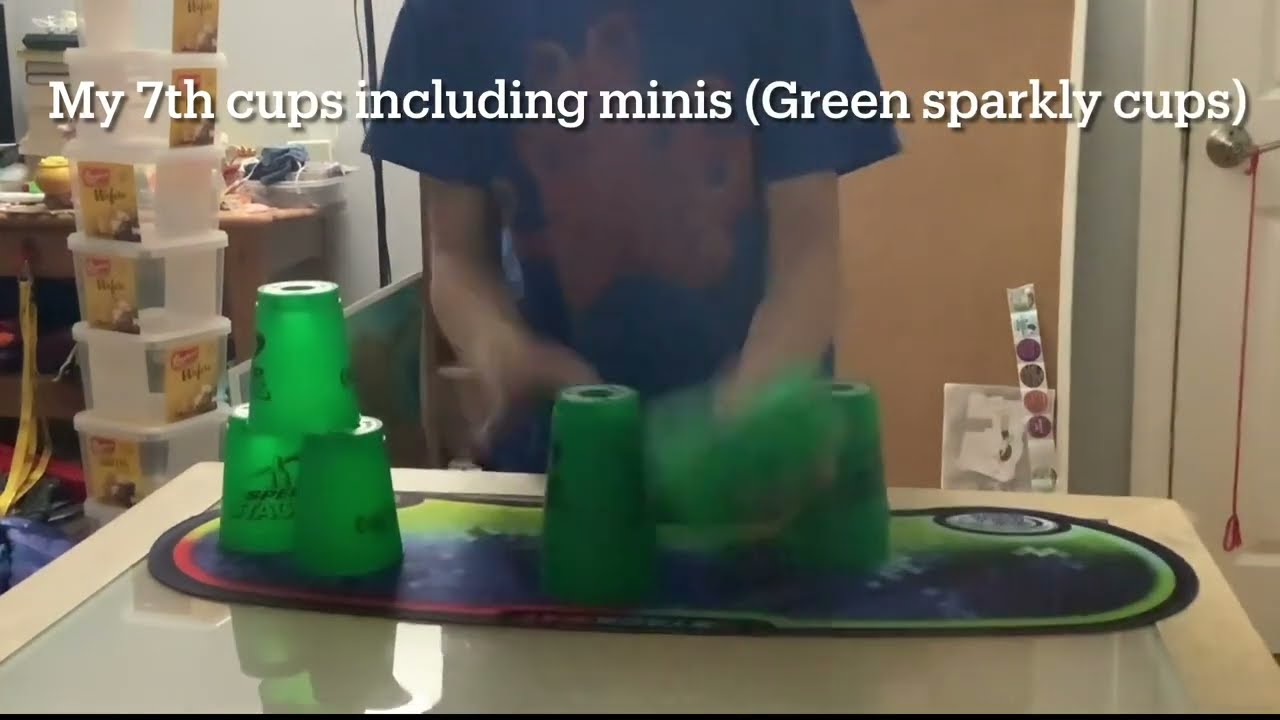In the image, a person is engaged in a cup stacking activity at a small, yellowish wooden table with a glass top surface. The individual, who appears to be a boy, is wearing a dark blue t-shirt adorned with a smeared, possibly red or brownish graphic design. His face is not visible; only his torso and arms can be seen. The table features a long, oval-shaped mat with a vivid and somewhat splotchy design that includes shades of blue, green, red, and black trim.

In front of the person, vibrant green plastic cups are being dynamically stacked. The left side of the table shows three cups arranged in a pyramid, while the right side shows two more cups, giving the impression that the stacking motion has caused some blur. An additional stack of clear plastic containers with yellow labels is visible in the background.

The scene is set against a backdrop of a brown wall, a white door on the right edge with a red string hanging from the doorknob, and a slightly cluttered table on the left side. Overlaying the top of the image is text in white font that reads, "My 7th cups including minis. Green sparkly cups."